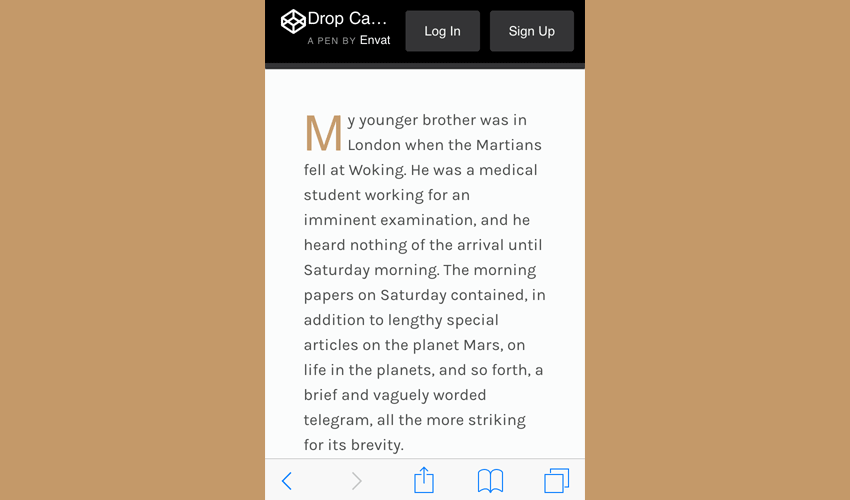The image features a predominantly grey background, punctuated by elements of brown on either side. Towards the left and right edges, patches of brown are noticeable, providing a frame for the central content. A subtle grey bar runs across the middle, dividing the image. 

Text elements are scattered throughout: "pin by invent," "log in," "sign up," are displayed prominently, accompanied by the word "order" in black. Another text, "brown M," stands out with a note about its brevity, making it particularly striking.

Navigation icons include a blue left arrow and a grey right arrow, enhancing the visual flow. Additional interface elements like a square with an up arrow, another square, and several other squares are present, adding to the layout's complexity.

Lastly, a small bug icon is included within the composition, hinting at a possible theme or focus of the visual content. Despite the assorted elements, the image maintains a cohesive color palette dominated by grey and brown tones.